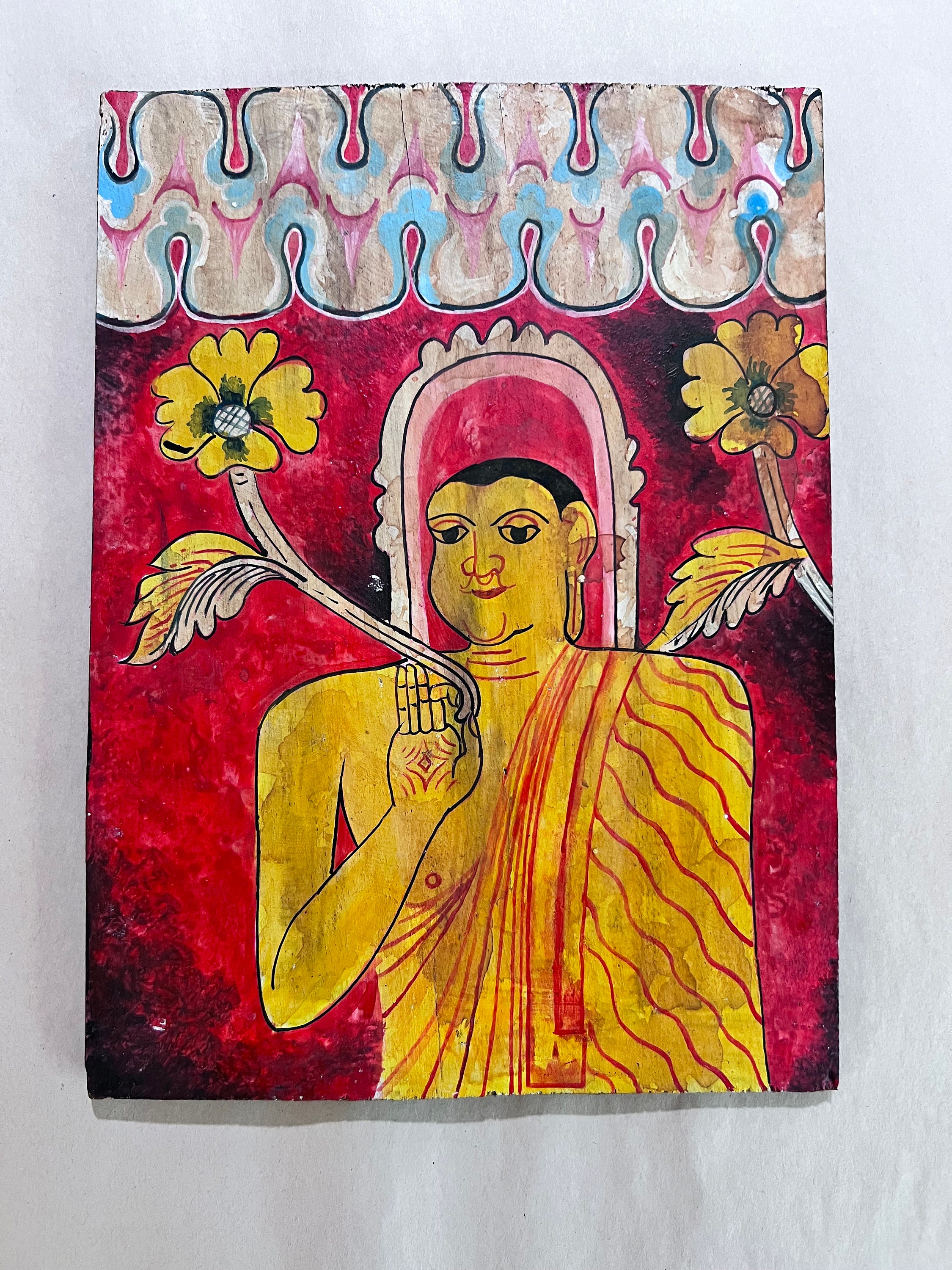The final image in the sequence features a detailed painting with a gray and whitish background, seemingly created using markers or watercolor. The composition starts at the top with small drips surrounded by black, transitioning to white and pink within. Below this, a squiggly line borders the piece, featuring white edges and shades of pink and blue in the middle. This upper section merges into a pink background, accented by black areas, particularly at the bottom left and right corners, and speckled around the composition.

Centrally, the painting depicts an abstract male figure. He has black hair, black eyes, red lids, and brows, with a red nose and mouth. His entire body is rendered in yellow, with an item in his hand and additional red details, like clothing. The man holds yellow flowers with white stems; the leaves show a dual color scheme—white on the back and yellow and red on the front. Encircling his head is a white area set against a pink background, resembling a mirror or reflective surface.

Additional elements suggest he might be seated or resting on a chair, with an exposed shoulder suggesting a toga-like garment. His pose hints at holding the flower with a hole in his palm, adding a layer of intrigue to the image. Overall, the artwork is saturated with reds and yellows, creating a striking visual impact on this rectangular canvas.